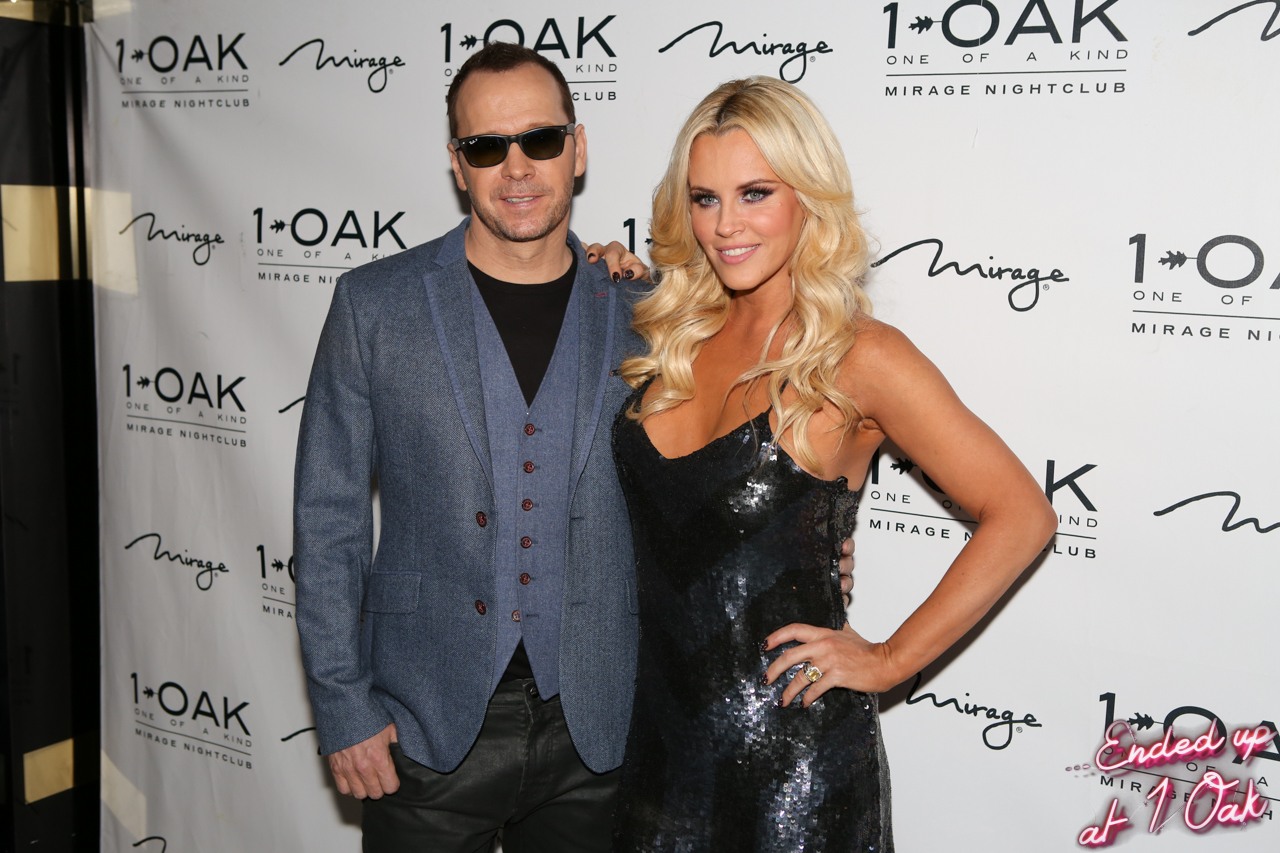In this photo, a celebrity couple stands in front of a promotional backdrop adorned with repeating logos for One Oak and Mirage Nightclub. The man, identified as Donny Wahlberg, a former boy band singer, is dressed in a light blue dress suit paired with a black undershirt, black pants, and black sunglasses. His right arm affectionately wraps around his date. She is a blonde woman, wearing a stylish black leather cocktail dress that sparkles under the lights. Behind them, the white banner features small leaf icons intertwined with the text "One Oak - One of a Kind" and "Mirage Nightclub" in black letters. In the lower right corner of the banner, the phrase "Ended Up at One Oak" is prominently displayed in white letters with a pink outline. Both individuals are looking directly at the camera, exuding confidence and elegance.